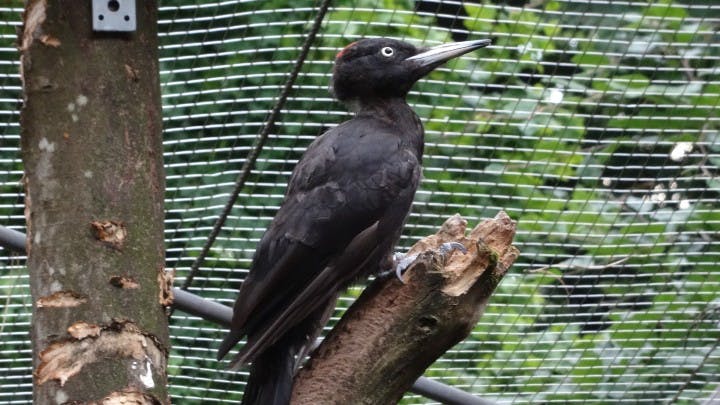A striking black bird with a few brown feathers on top and a dash of orange on its forehead is perched on a broken wooden branch in what appears to be a bird habitat. The bird, identified as likely a woodpecker, has its head turned slightly up and to the right. Its white beak, which fades to black at the tip, complements its white eyes with dark pupils. The bird’s wings feature feathers that point directly downward, and its claws grip the light-colored broken part of the branch, which contrasts with the darker brown of the rest of the tree limb. Behind the bird, a thick, silver metal grid fence provides a backdrop, suggesting a caged environment. To the left of the bird, a partially notched tree trunk, tinged with green, extends upwards, topped with a metallic square bracket punctuated by three holes. The background beyond the metal screen appears to be lush with greenery, and there are faint hints of other birds among the blurred foliage.